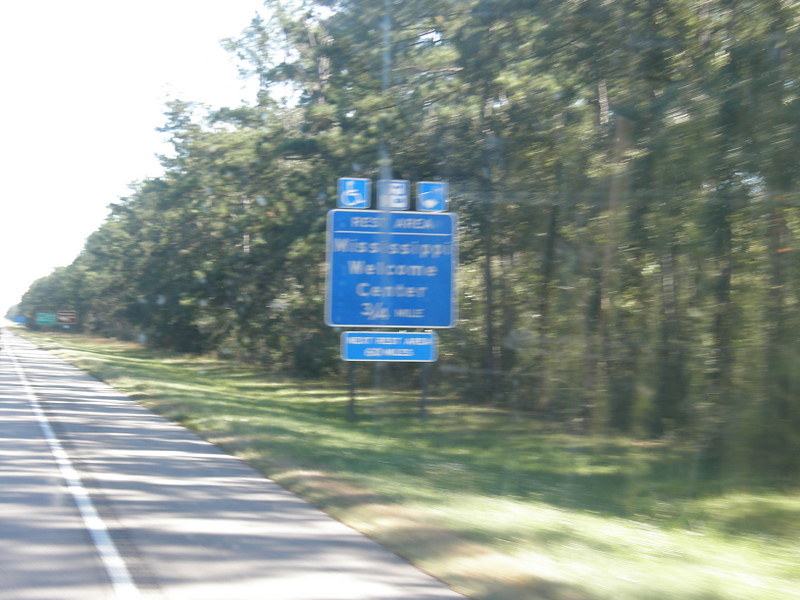This photograph, taken from a moving car, is slightly out of focus. In the bottom left corner, there is part of the road, along with the shoulder and the verge separating them. The image captures the side of the road where a grassy area extends into a line of trees that runs from the right side towards the left background. At the center of the photograph, a rest area sign stands prominently, reading "Mississippi Welcome Center, 3/4 Mile." Although blurry due to the motion, the sign also includes smaller text below that likely indicates "Next Rest Area, 60 Miles." Additionally, the sign features various icons, including one denoting wheelchair accessibility, while the others are indistinct.